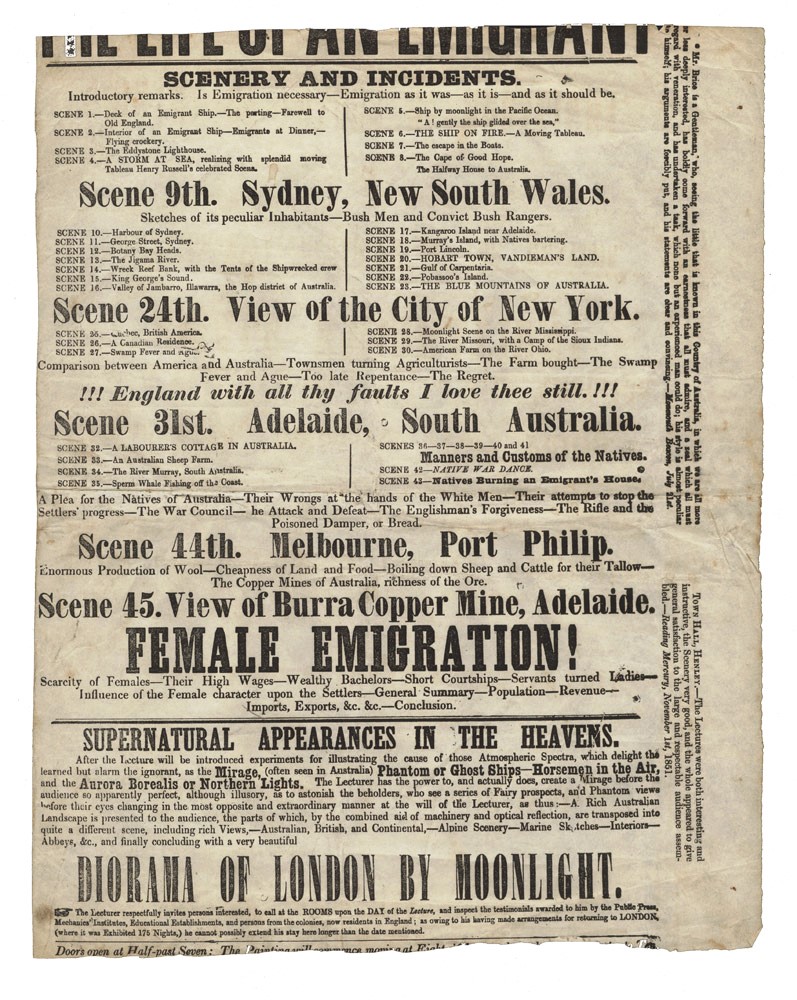This image depicts a vintage newspaper cutout, characterized by its discolored, aged appearance with a mix of whitish, grayish, and tan hues, and featuring black ink text. The header at the top prominently displays "Scenery and Incidents." Below, several numbered scenes are listed, starting with "Scene 9: Sydney, New South Wales," followed by "Scene 24: View of the City of New York," "Scene 31: Adelaide, South Australia," "Scene 44: Melbourne, Port Phillip," and "Scene 45: View of Burra, Cooper, Mine, Adelaide." Additional sections mention topics like "Female Immigration," "Supernatural Appearances in the Heavens," and "Diorama of London by Moonlight." The layout suggests the scenes and topics might be part of a larger narrative or play, giving the newspaper a richly historical and theatrical flavor.